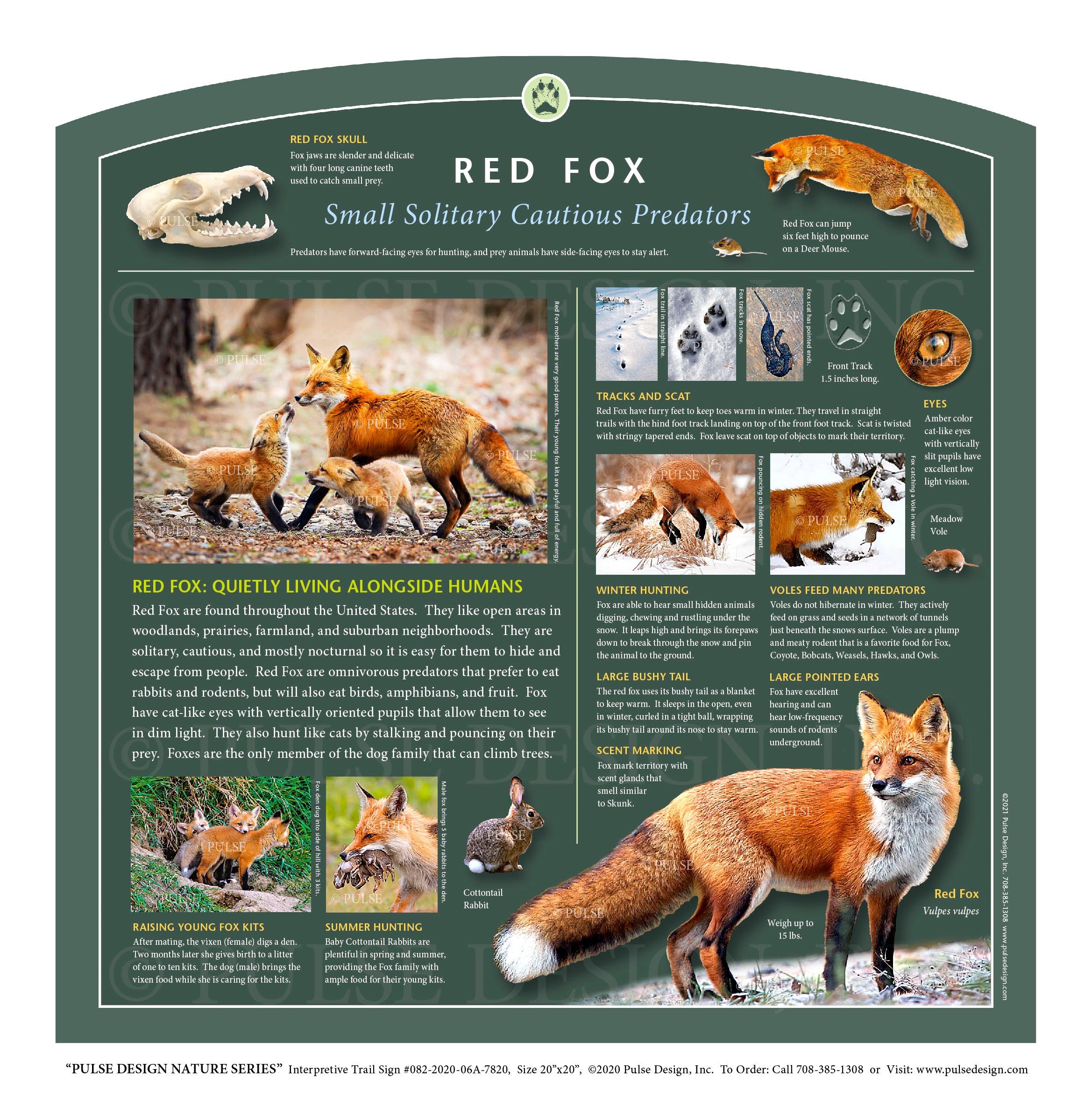This is an interpretive trail sign from the Pulse Design Nature Series, typically found in parks, national forests, or educational environments. The sign, which features a green background with an arched top and a round logo of a paw print, is dedicated to the Red Fox. The top of the sign is labeled with "Red Fox: Small, Solitary, Cautious Predators."

The sign includes a detailed infographic, starting with a photograph of a fox skull on the top left and a red fox poised to pounce on the top right. In the central section, there is a full-grown fox standing majestically and a photograph of a mother fox with two kits, illustrating family life.

Text on the sign explains that red foxes live quietly alongside humans and are found throughout the United States. Preferred habitats include open areas like woodlands, prairies, farmlands, and suburban neighborhoods. As mostly nocturnal and solitary animals, they are cautious and skilled at hiding and escaping.

The red fox is described as an omnivore that primarily preys on rabbits and rodents but also consumes birds, amphibians, and fruit. They uniquely possess cat-like eyes with vertically oriented pupils, aiding in low-light vision, and they hunt by stalking and pouncing. Remarkably, foxes are the only members of the dog family that can climb trees.

Additional visuals and text describe their behaviors and physical characteristics: during summer and winter hunting, raising young fox kits, tracks and scat, and scent marking. Highlighted are features like their large pointed ears and bushy tails.

The bottom of the sign includes the Pulse Design Nature Series credit, contact information, size, and copyright details, giving it a professional and informative finish.